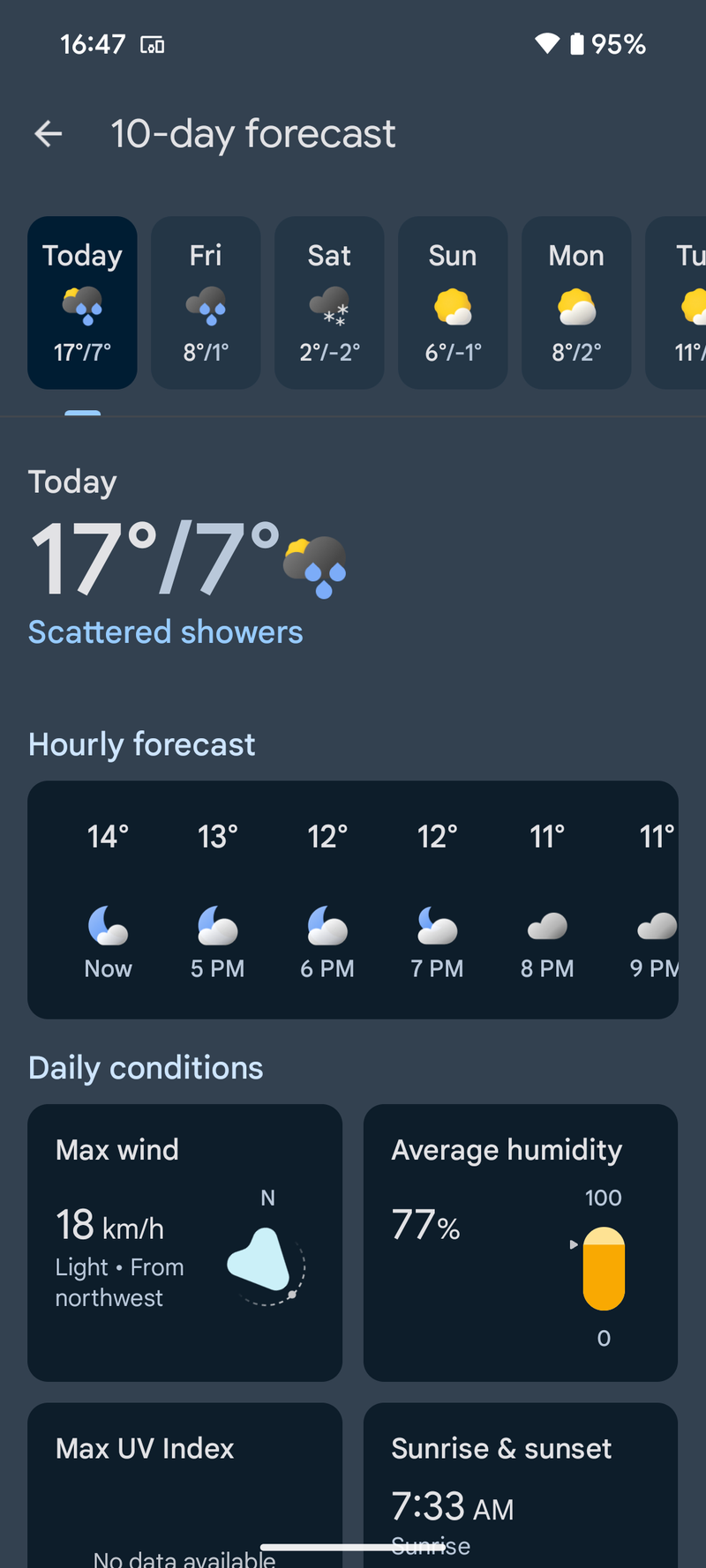In the image, we see a detailed weather app interface, typical of one you might check on your smartphone. The status bar at the top shows it is currently 16:47 in military time. The device's battery level is at 95%, with full signal strength indicated by the icon to the right.

The search term entered was for a 10-day forecast, clearly visible at the top of the forecast section. The forecast information is presented with specific days: today, Friday, Saturday, Sunday, Monday, and Tuesday. However, only today's and the first few days' forecasts are fully visible.

For today, the high temperature is 17°C, with a low of 7°C, and scattered showers are expected. The following days’ temperature highs and lows are listed as:
- Friday: High of 8°C, Low of 1°C
- Saturday: High of 2°C, Low of -2°C
- Sunday: High of 6°C, Low of -1°C
- Monday: High of 8°C, Low of 2°C
- Tuesday: Partial display showing a high of 11°C

The hourly breakdown for the evening is included, showing temperatures of 14°C at 5 p.m., 13°C at 6 p.m., 12°C at both 7 p.m. and 8 p.m., and 11°C at 9 p.m. Winds will reach a maximum speed of 18 kilometers per hour, and the average humidity is noted as 77%. Although some details are partially cut off, the sunrise is listed at 7:33 a.m., and there is a reference to a max UV index.

Overall, the app provides a comprehensive view of the current weather conditions and the upcoming forecast.